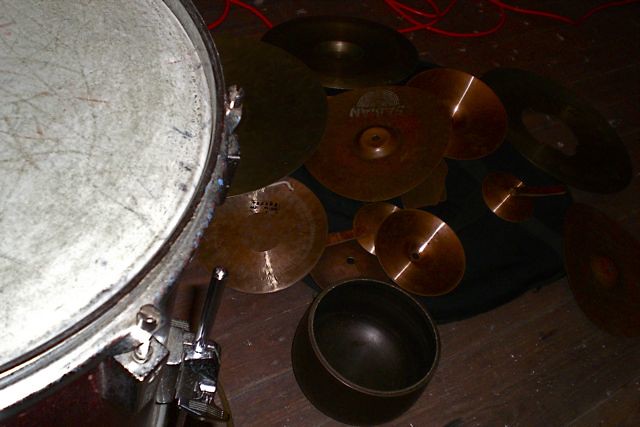The photograph captures an intricate scene of a disassembled drum set, taken from an unusual angle as if standing behind the drums. The left side of the image prominently features a tom-tom drum with a well-used, grayish-white drumhead, marked by extensive brown and gray scratches and a slightly visible silver edge. The reddish-brown side of the drum adds to its weathered look. Dominating the center of the image, a collection of shiny, goldish-bronze cymbals lies scattered in an overlapping manner on a worn, dark brown wooden floor. The cymbals, reflecting the camera’s light, feature varying sizes and are not neatly piled but rather spread around in a disarray. The scene also includes a disassembled drummer's throne, indicating the drum set is either being assembled or disassembled. The composition is framed against a deep brown background, with a glimpse of red wire hanging at the top, further adding to the sense of a setting in transition.